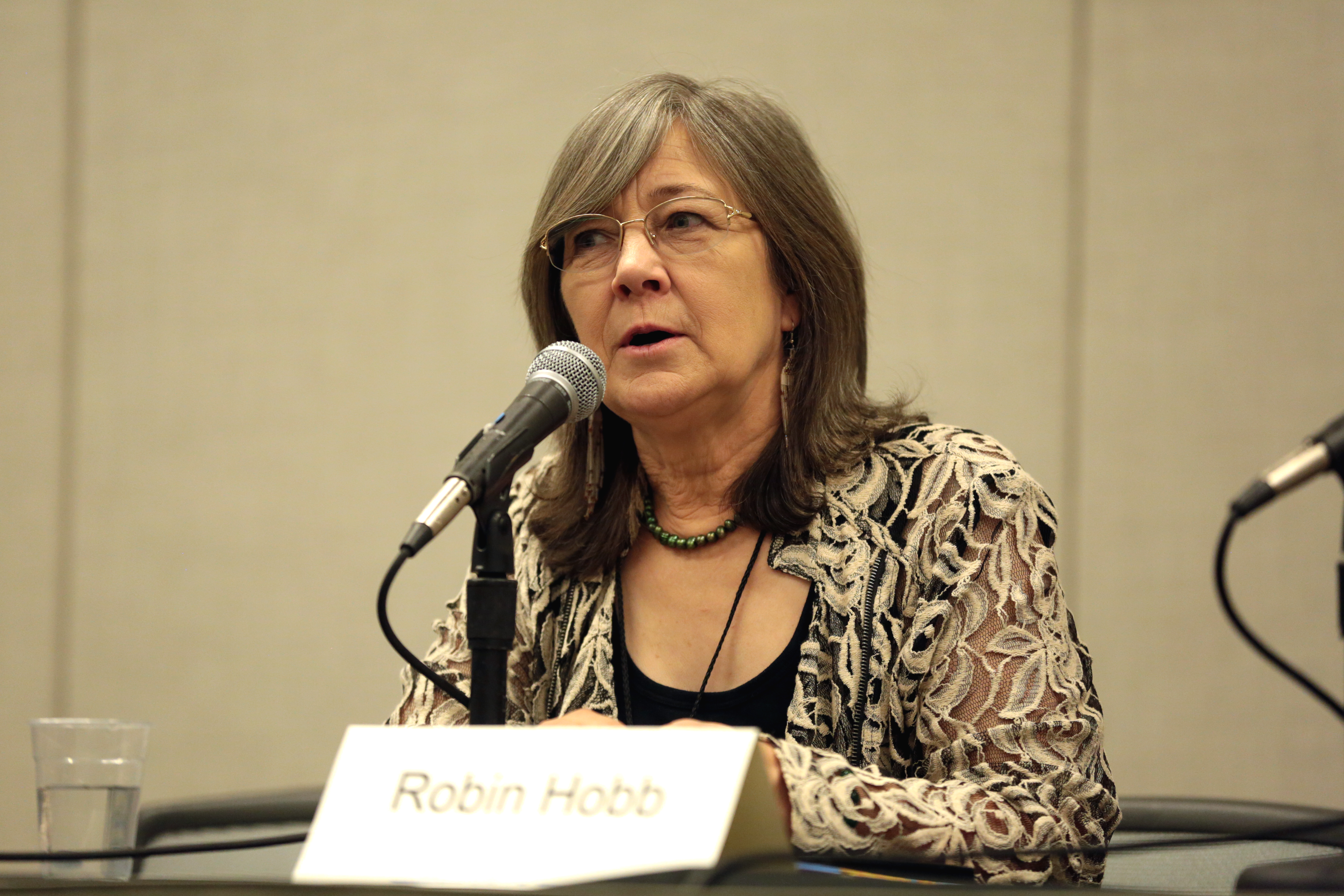The photographic image captures a 50-year-old woman, Robin Hobb, indoors against an off-white wall. Her shoulder-length gray hair is parted to her left, and she wears oval rimless glasses. She is slightly tilting her head and speaking into a desk-mounted black and gray microphone. Robin's attire includes a brown floral print long-sleeve shirt over a brown tank top, complemented by a green beaded necklace close to her neck. Around her neck is also a black string, part of an unseen shoulder bag. In front of Robin, a folded piece of paper bears her name, "Robin Hobb" in black text. A glass of water, about two-thirds full, is positioned to her right. Behind her is an off-white wall with subtle vertical lines.